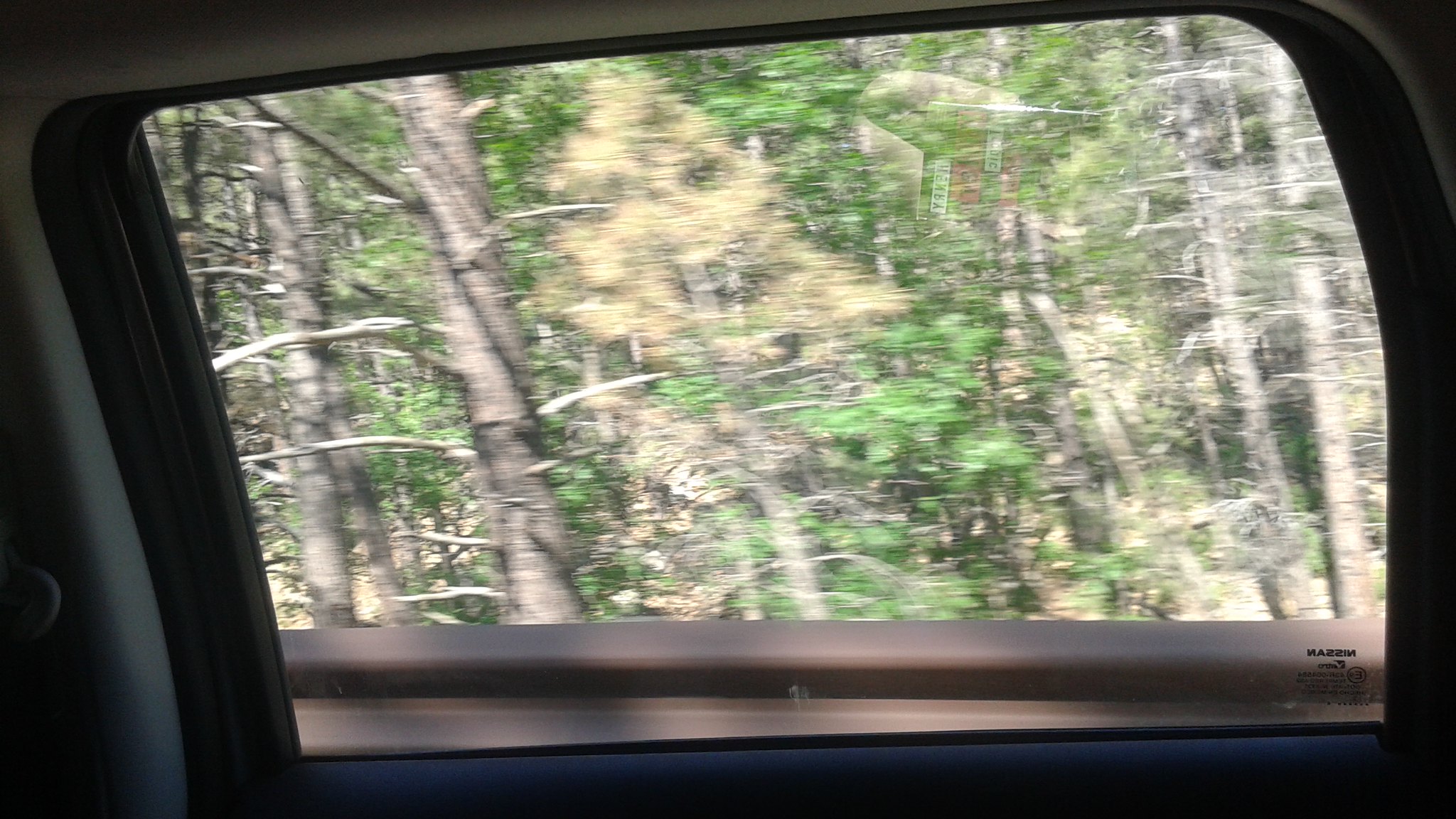The photograph captures a slightly blurred view from the passenger side of a moving car, possibly due to the car's speed or camera quality. Inside the car, the interior features a gray color scheme with a black rubber lining around the window frame, and a slightly darker trim below the window. Looking out, a brown steel guardrail lines the edge of the road. The passing landscape includes several trees varying in trunk thickness, some with branches shooting off. The trees predominantly have green leaves, although some leaves appear yellow or brown, possibly on a dying tree. In the center of the view, there's a grassy, hill-like area devoid of trees.